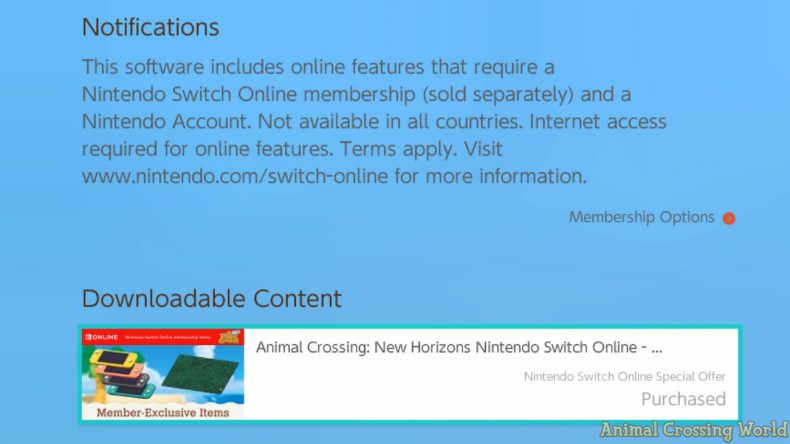This is a meticulously edited promotional image highlighting various features and membership options for Animal Crossing: New Horizons with a Nintendo Switch Online subscription. In the bottom right corner, a white watermark stating "Animal Crossing World" is visible. The image is primarily dominated by textual information.

At the top, bold black letters spell out "Notifications." Just below, a detailed notice informs users that "The software includes online features that require a Nintendo Switch Online membership, which is sold separately, along with a Nintendo account. Furthermore, these features are not available in all countries, and internet access is required. Terms apply. For more information, visit www.nintendo.com/switch/online."

Further down, the section titled "Membership Options" is prominently displayed, emphasized by a red dot edited onto the photo to draw attention to this area. 

In the bottom left corner, another header in bold black letters reads "Downloadable Content." To the left of this section, it mentions a "Member Exclusive Item" and showcases a photo of the Animal Crossing game alongside a Nintendo Switch advertisement. To the right, the text reads "Animal Crossing: New Horizons Nintendo Switch Online."

Finally, in the bottom right corner, the image includes a mention of a "Nintendo Switch Online Special Offer Purchased."